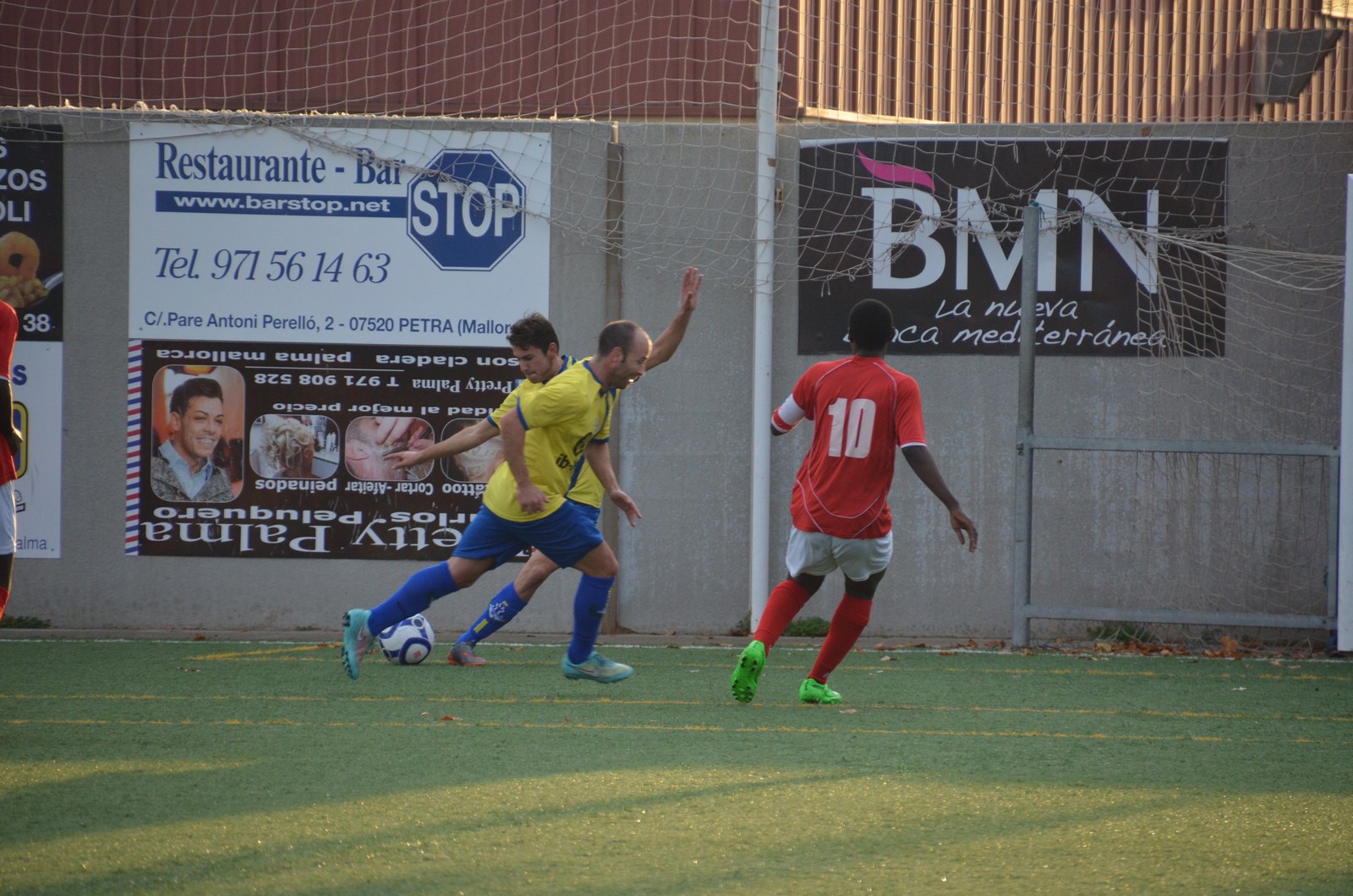This image captures a lively soccer match featuring three men on an aged green field with faint, faded yellow stripes. In the foreground, two men are wearing yellow jerseys paired with blue shorts and blue socks. Both players are in motion, with one appearing prepared to kick the soccer ball while the other, who is balding and older, advances alongside. Positioned to the right, with his back towards the viewer, a third player wears a red jersey emblazoned with the number 10 in white, red socks, and green tennis shoes. This player has darker skin, adding to the diversity on the field.

The background reveals a setting enclosed by a light tan or gray concrete wall adorned with several banners. Centrally, a white pole stretches upwards, dividing the visual space. Prominent among the banners is a white one advertising a "Restaurante-Bar" along with a phone number and other details. Adjacent to it, a black banner with white lettering stands out, reading "BMN" in Spanish. Above the concrete barrier, a reddish sheet metal wall is partially visible, adding an industrial touch to the scene. This carefully detailed setting suggests an urban environment where enthusiasm for soccer brings people together.